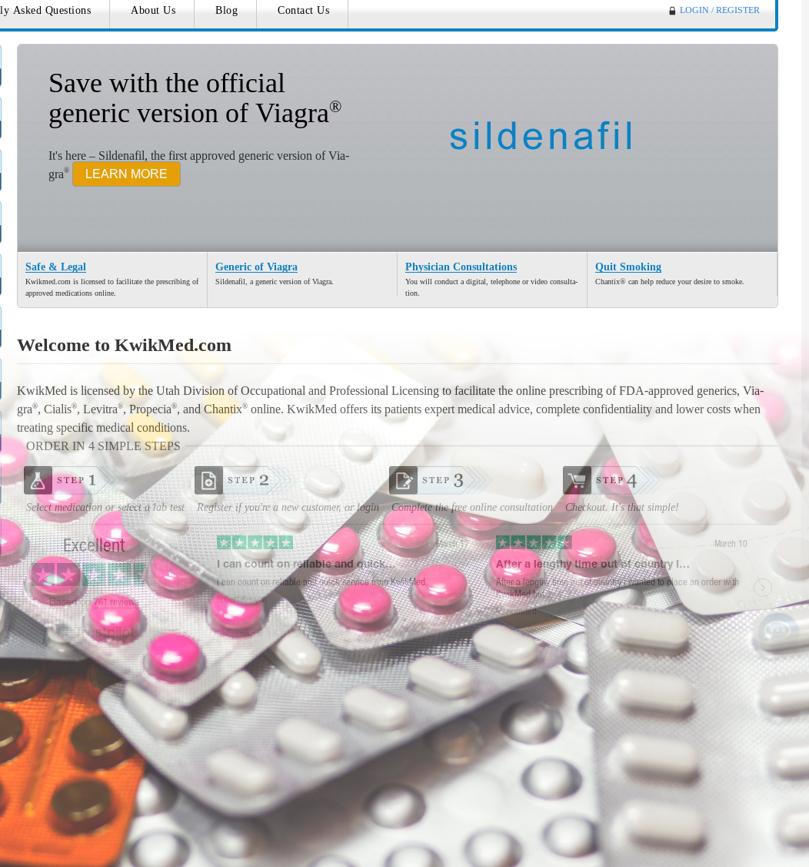This vibrant and visually engaging image showcases a partially visible website, where the top navigation bar displays tabs for "Ask Questions," "About Us," "Blog," "Contact Us," and a blue text link for "Login/Register." The right side features a prominent banner announcing "Save with the Official Generic Version of Viagra," with a subtext introducing "Sildenafil," the first approved generic version. Adjacent to this banner is a yellow "Learn More" button and the word "Sildenafil" highlighted in blue. 

Below this header section, the image is divided into four clickable links with brief descriptions:
1. "Safe and Legal" - QuickMed is licensed to prescribe approved medications online.
2. "Generic of Viagra" - Information about Sildenafil, the generic version of Viagra.
3. "Physician Consultations" - Options for digital, telephone, or video consultations.
4. "Quit Smoking" - Details on Cherox, which aids in reducing the desire to smoke.

Further down, "Welcome to QuickMed" introduces the company, detailing its licensing by the Utah Division of Occupational and Professional Advising to prescribe FDA-approved generics such as Viagra, Cialis, Levitra, Propecia, and Chantix. QuickMed offers expert medical advice, complete confidentiality, and cost-effective treatment options for specific medical conditions.

The site also outlines an easy four-step process for ordering:
1. Select medication or lab test.
2. Register if you're a new customer.
3. Complete the free online consultation.
4. Check out - it’s that simple.

The background under the "Welcome to QuickMed" section is adorned with an assortment of colorful pills, including white and pink ones. However, the text here is somewhat hard to read due to the busy background.